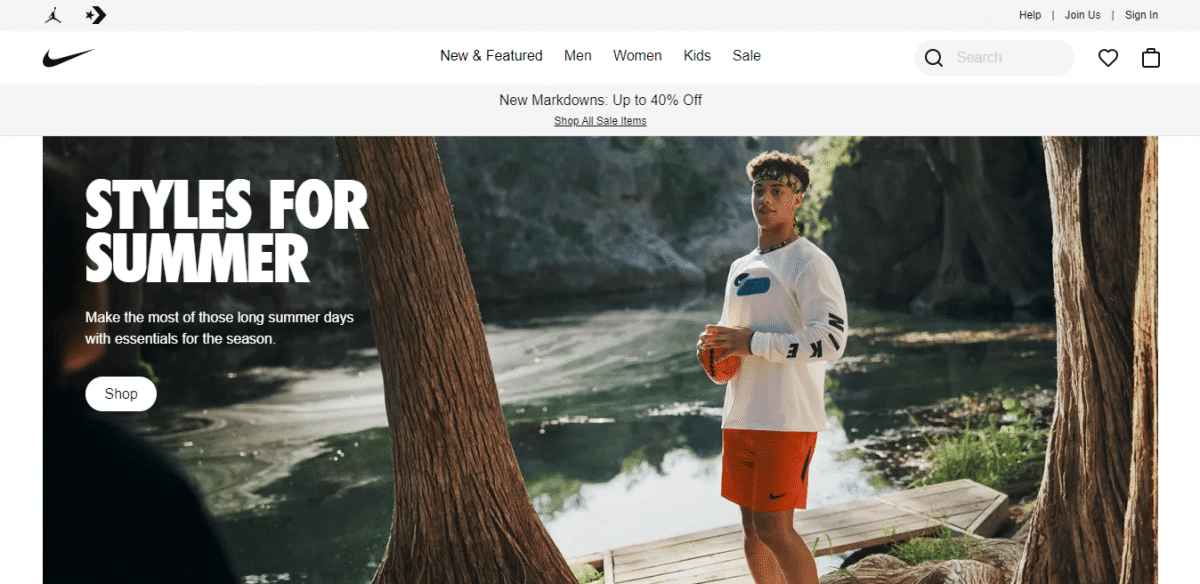This is a Nike webpage showcasing their products. In the top right corner, the options "Help," "Join Us," and "Sign In" are prominently displayed. Below these links and to the left against a white background is the iconic Nike logo. The navigation menu features categories such as "New & Featured," "Men," "Women," "Kids," and "Sale." Adjacent to these categories is a search box labeled with the word "Search," followed by icons of a heart and a briefcase.

Beneath the navigation bar, against a gray background, an announcement reads, "New Markdowns, Up to 40% Off. Shop All Sale Items." Below this text is a large, eye-catching photo. The main subject of the photo is a young man outdoors, standing in front of a body of water that appears to be a river or stream. He is wearing a long-sleeve white shirt with "Nike" emblazoned on the visible left sleeve, complemented by a headband. He is holding an orange object, likely a football, and is dressed in orange shorts that also feature the Nike logo.

The background of the image includes the water, trees, and possibly some rocks, although it is slightly blurry. In the foreground, a tree trunk is present to the far right, another tree trunk is beside the young man, and a possible third tree trunk is on the far left. The photo is accompanied by text that reads, "Styles for Summer. Make the most of those long summer days with essentials for the season. Shop."